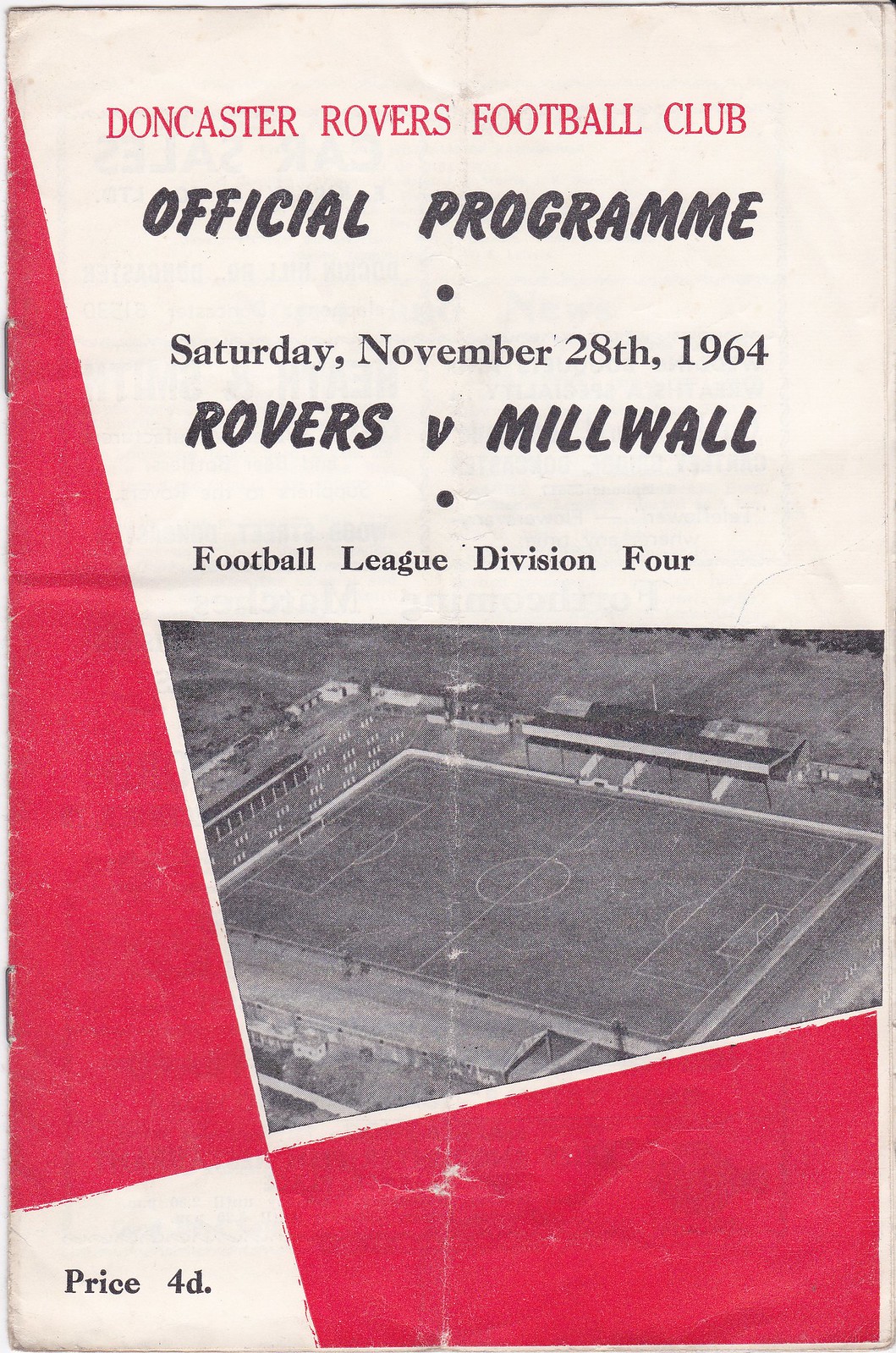This detailed caption provides a comprehensive description of the front cover of a football program:

This is the front cover of the official program for Doncaster Rovers Football Club. The top of the pamphlet prominently displays the title "Doncaster Rovers Football Club Official Program" in red, with a small dot circle beneath it. Below the circle, the date "Saturday, November 28th, 1964" is printed. Further down, "Rovers v. Millwall" is indicated, followed by another dark circle, and then "Football League Division IV."

The program features a black and white photograph at its center, showcasing an aerial view of a stadium. The image reveals the field's white out-of-bounds lines, grandstands on both sides, and a scoreboard situated behind the left goal. Red triangles adorn the right and left corners of the cover. The bottom section reads "Price 4D" on the left side. The cover's design integrates white with red and black accents, creating a visually striking appearance.